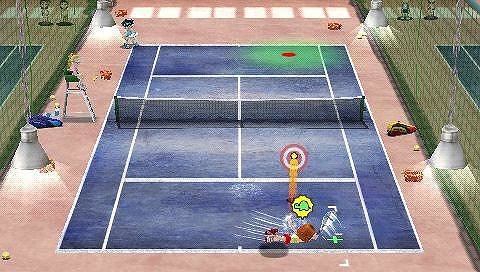The image is a detailed screenshot from a tennis-themed video game. It showcases a vibrant court scene where characters are actively engaged in a match. The court itself is blue with distinct white lines marking the boundaries, while the area surrounding it is painted a vivid pink. Overhead, four lamps illuminate the scene from the ceiling, suggesting the setting is indoors. 

In the foreground, a player is captured in an intense moment, diving to the right with a racket in hand, accompanied by a small turtle icon above their head. This player appears to be making an attempt to hit a ball, which is marked with a bullseye symbol. Left of the screen, a person sits on a green chair, observing the game. 

On the upper part of the court, another character, possibly dressed in a blue shirt, stands poised, ready for the next move. Scattered around the ground are several tennis balls and a couple of tennis bags, adding to the realistic yet cartoonized environment of this well-detailed game scene. The entire area seems to be outlined by nets, encapsulating the court, and adding to the competitive atmosphere of this engaging sports simulation.